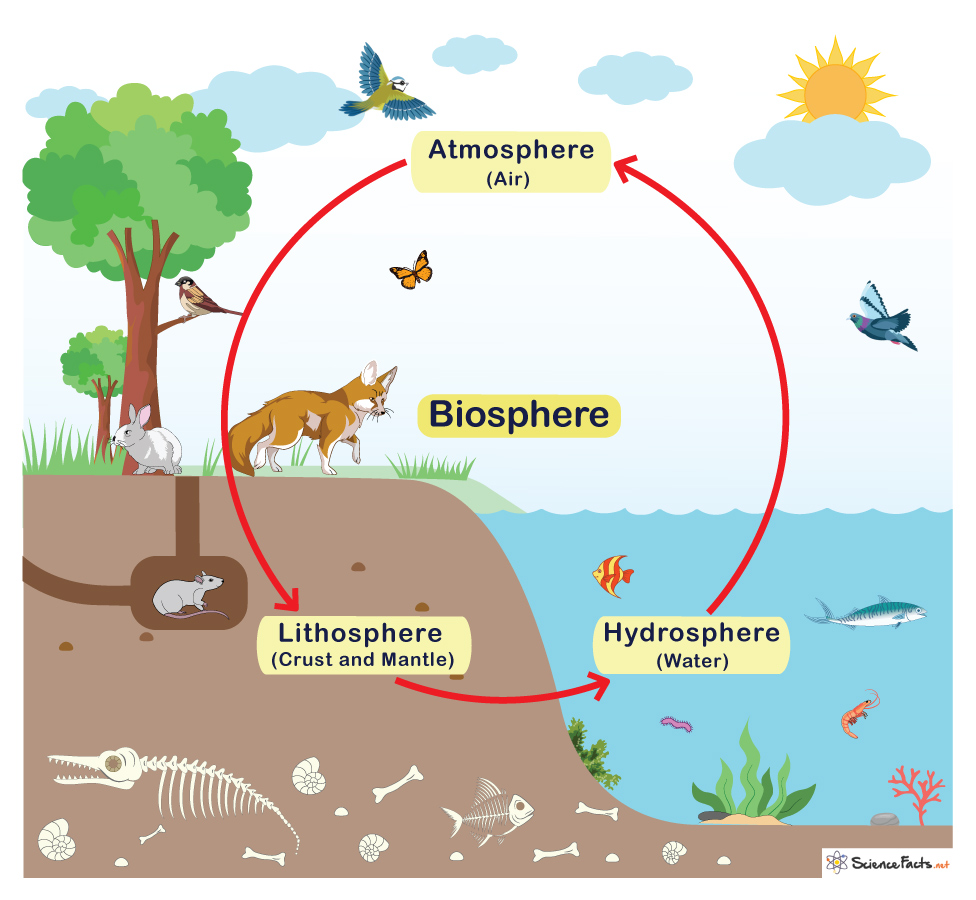This is a detailed, computer-animated, square diagram labeled "Biosphere," illustrating the interactions between various Earth systems. The background is completely white, which contrasts with the colorful elements within. The diagram showcases three main labeled regions: the atmosphere (sky), the lithosphere (earth), and the hydrosphere (water). In the upper left, there's a prominent green tree with another in the background, while a vibrant yellow sun and a bird flying are positioned in the upper right. Blue clouds partially fill the sky, adding depth.

A significant red circle with counterclockwise arrows runs through the center of the image, outlining the interconnected nature of these Earth systems. Inside this circle, "lithosphere" is labeled over the land, with "crust and mantle" in parentheses, "hydrosphere" is marked over the water with "water" in parentheses, and "atmosphere" at the top with "air" in parentheses. A fox, a bunny, and a bird sitting on a branch represent the terrestrial fauna, while a pair of swimming fishes occupy the depicted pond waters.

Beneath the surface, the dirt area hosts detailed elements such as fossils and a small brown animal, likely a mole or rat, residing in a dug hole. The image is completed in a cartoon-like graphic style, illustrating the cycle of life and the harmony between different ecological zones. The lower parts of the diagram dwindle into the earth, curving from the left to the right, depicting more details about life below the surface.